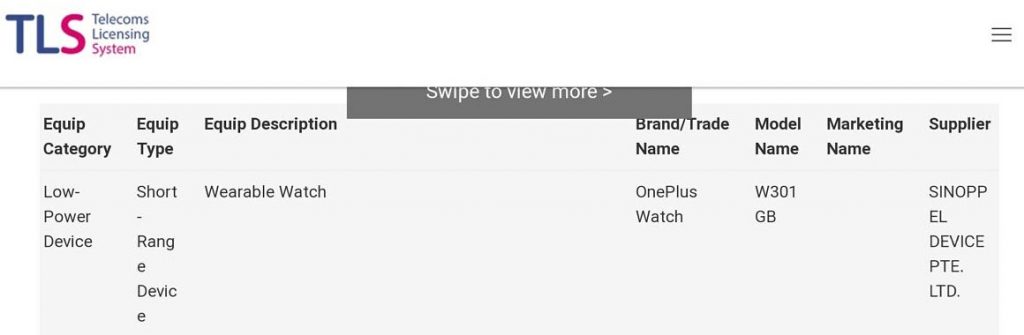This image appears to be a somewhat awkwardly cropped or scrolled-down screenshot displaying a data table. At the top, there's a frozen header, which presumably stays in place as one scrolls. The header includes the capitalized "TLS" logo, where the "S" is highlighted in pink. Next to the logo, the words "Telecoms," "Licensing," and "System" are stacked vertically, with "System" also in pink.

Below the header, the table presents detailed information about a piece of equipment. Here is the breakdown of the data provided:

- **Equipment Category**: Low Power Device
- **Equipment Type**: Short Range Device
- **Equipment Description**: Wearable Watch
- **Brand/Trade Name**: OnePlus Watch
- **Model Name**: W301GB
- **Marketing Name**: (left blank)
- **Supplier**: CINOPPEL (C-I-N-O-P-P-E-L, all in capital letters)
- **Device**: P-T-E. L-T-D. (also in capital letters)

The table is basic, with two columns: one for titles and another for corresponding results. Due to some awkward formatting, the columns appear quite narrow, causing the text to be cramped and somewhat difficult to read.